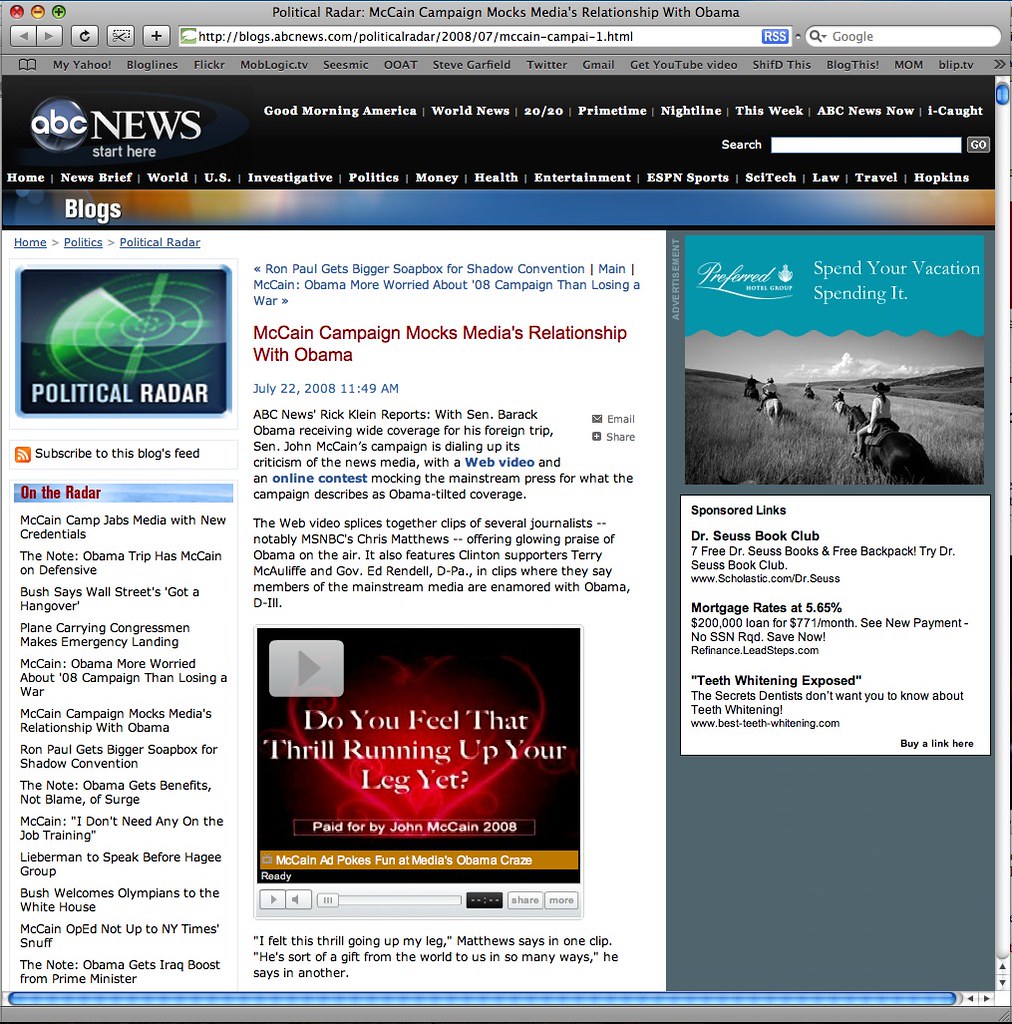The image captures a screenshot of a web page from ABC News. Dominating the top is a large black rectangular banner that prominently features navigation links for various sections such as Good Morning America, Weird News, 20/20, Primetime, This Week, and ABC News itself. Below this banner is another rectangular strip offering menu choices including News Brief, World, Money, Entertainment, and ESPN Sports.

On the left side of the page, there is a large white rectangular area. This section contains two notable images. The first image, located in the upper left-hand corner, is a visual depiction of radar accompanied by the text "Political Radar" just beneath it. In the lower right-hand corner of this same white rectangle, there is a video thumbnail with the caption, "Do you feel that thrill running up your leg yet?" This thumbnail features a red overlay with a large play button.

Within this white rectangular section, specifically in the first column, there is a list of political articles that users can access. The main headline in this column reads, "McCain Campaign Mocks Media Relationship with Obama," followed by several paragraphs of detailed information.

On the right-hand side of the webpage, there are two smaller squares stacked vertically. The top square is an advertisement for a hotel or resort, distinguished by an aqua header that reads, "Spend Your Vacation Spending It." Below this advert is another white square labeled "Sponsored Links," featuring promotional content for a Dr. Seuss book club, mortgage rates at 5.85%, and information on teeth whitening products.